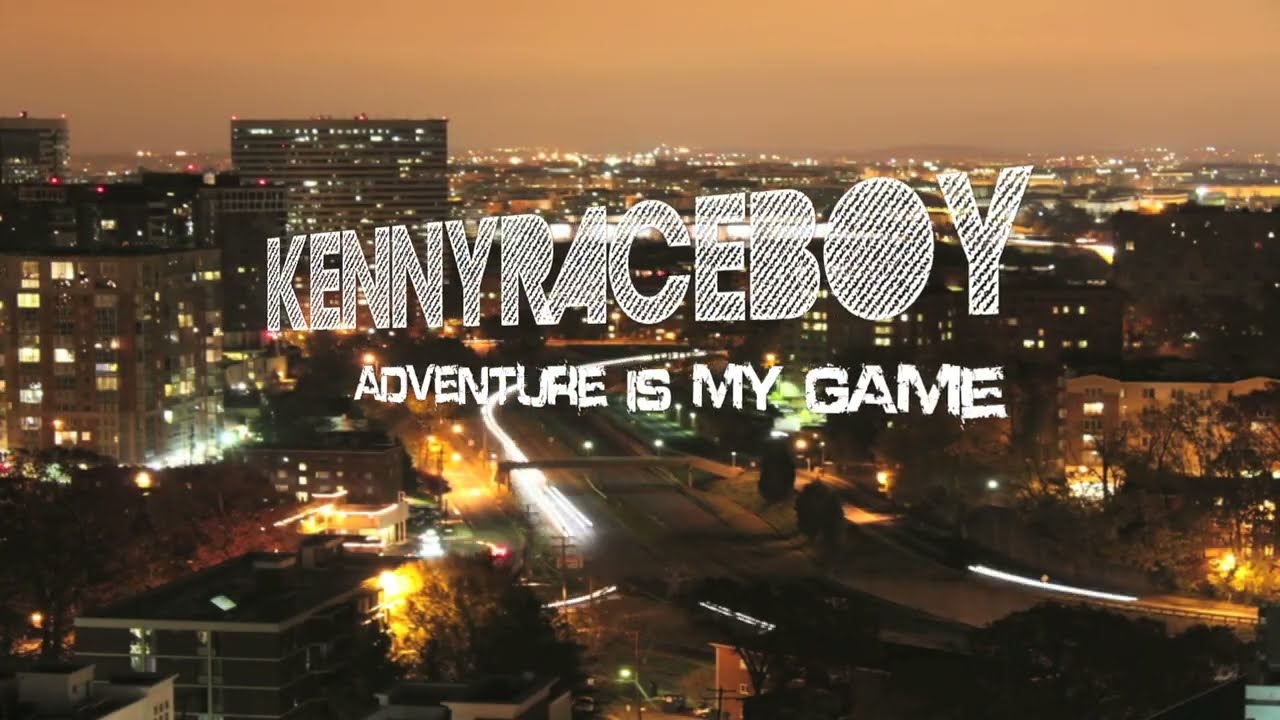In this image, we see a first-person view as if riding a blue motorcycle through a forested area. The motorcycle's front, showcased prominently, features a small windshield and a rear-view mirror on the left side. The bike's body is dual-toned with a darker blue on top and a lighter blue below. You can also see various gauges and meters on the dashboard. The scene unfolds on a rugged, dirt two-track road with numerous small rocks and pebbles scattered across it. On either side of the road, green trees and shrubs, some with brown trunks and green leaves, rise up, creating a dense forestry feel that extends into the distance. Above, the sky is a vibrant blue with white clouds drifting by, adding a sense of openness to the otherwise enclosed, green surroundings.